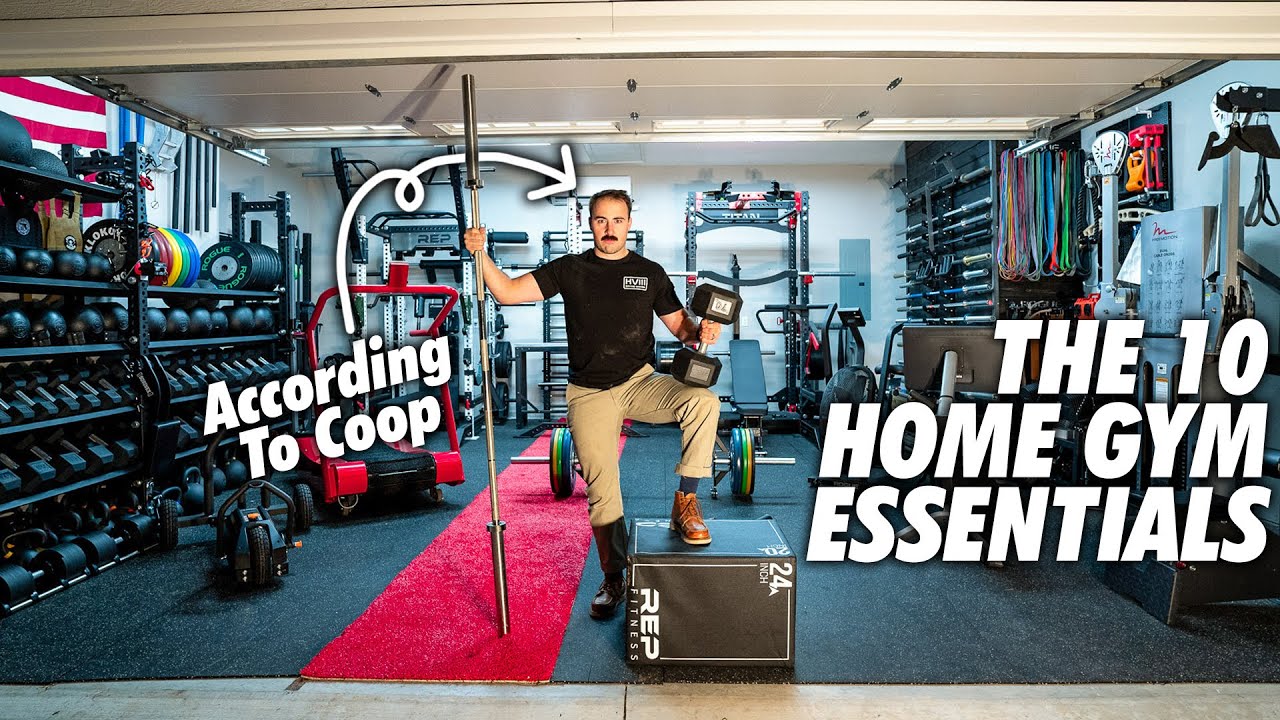The image depicts an elaborate, well-equipped home gym set up in a converted garage with a white back wall, identifiable by the visible garage door at the ceiling. Dominating the left side are two substantial metal shelving units loaded with a variety of hand weights, barbells—featuring circular, square, and cylindrical ends—and additional heavy lifting weights. A red treadmill sits prominently in the foreground with an unidentified machine directly behind it, adjacent to a climbing ladder and a weightlifting machine. An exercise bike is positioned in front of these machines.

On the right wall in the background, several weighted pulling straps and numerous plastic pull straps for exercising are organized. A red runner carpet spans from the front to the back of the gym area. The focal point of the image is a man, presumably Coop, standing confidently in the center. He is dressed in khaki pants and a gray shirt with a mustache, holding a barbell in his left hand and a weightlifting pole in his right hand. His left foot is propped up on a small platform marked "24 Rep Fitness." Text across the image reads "10 Home Gym Essentials According to Coop," with an arrow pointing to him. An American flag adorns the left wall, adding a patriotic touch to the detailed setup. The scene serves as an advertisement or a YouTube video thumbnail highlighting essential home gym equipment curated by Coop.